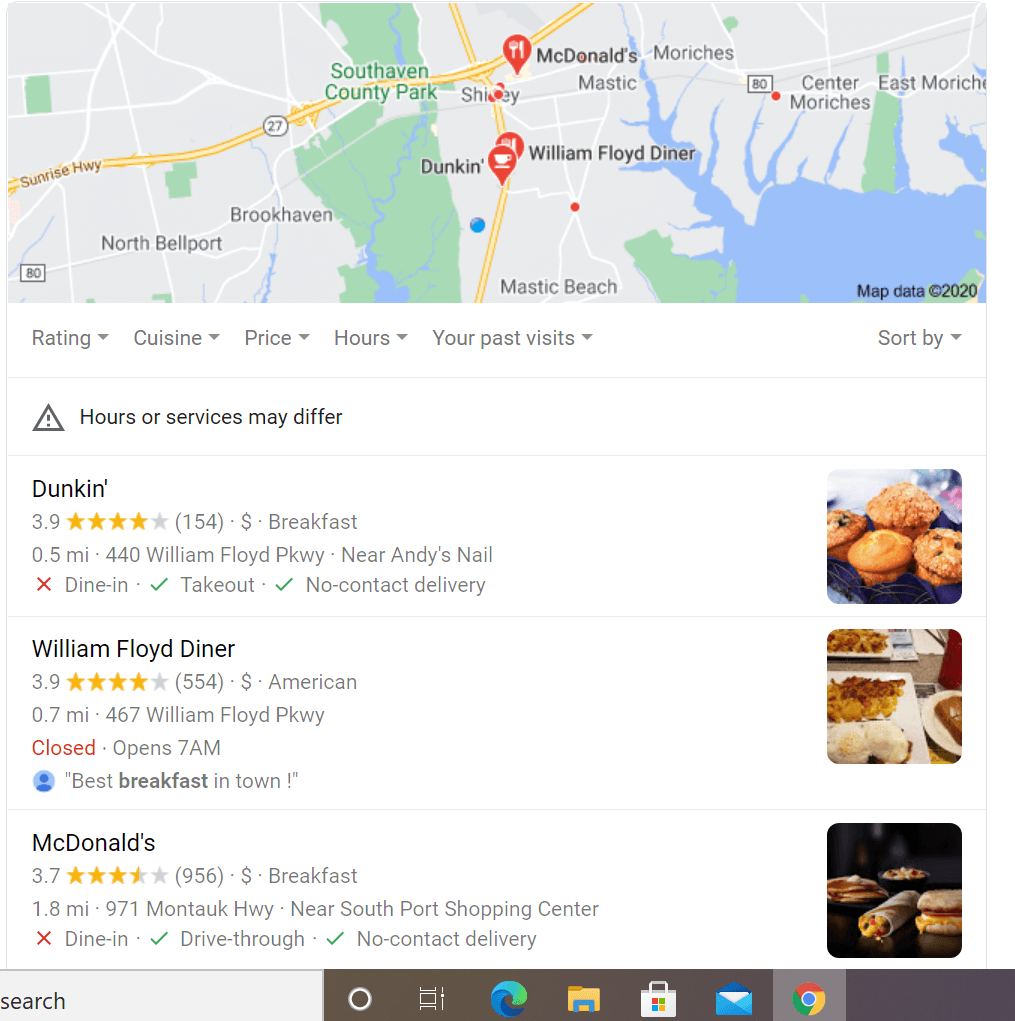A user is viewing Google Chrome, as indicated by the highlighted Chrome icon at the bottom of the screen. The browser is displaying a version of Google Maps. At the top, search results include locations such as McDonald's and William Floyd Diner. 

Below these, there are light gray menu options for sorting by rating, cuisine, price, hours, and past visits; each with a downward-pointing triangle indicating drop-down menus. On the right, options can be sorted with another drop-down menu, marked by an upside-down triangle. A dark gray triangle with an exclamation point notifies that "hours or services may differ."

The first listing is for Dunkin', showing a 3.9-star rating from 154 reviews. Five stars are displayed, with one star gray, indicating a near-four-star rating. There is an image of muffins: a corn muffin, a possible maple muffin, a chocolate chip muffin, and a blueberry muffin.

The next listing is William Floyd Diner, rated 3.9 stars from 554 reviews. It is located 0.7 miles away at 467 William Floyd Parkway. The image shows an assortment of pastries or breakfast items on tables.

The final listing is McDonald’s, with a 3.7-star rating from 956 reviews.